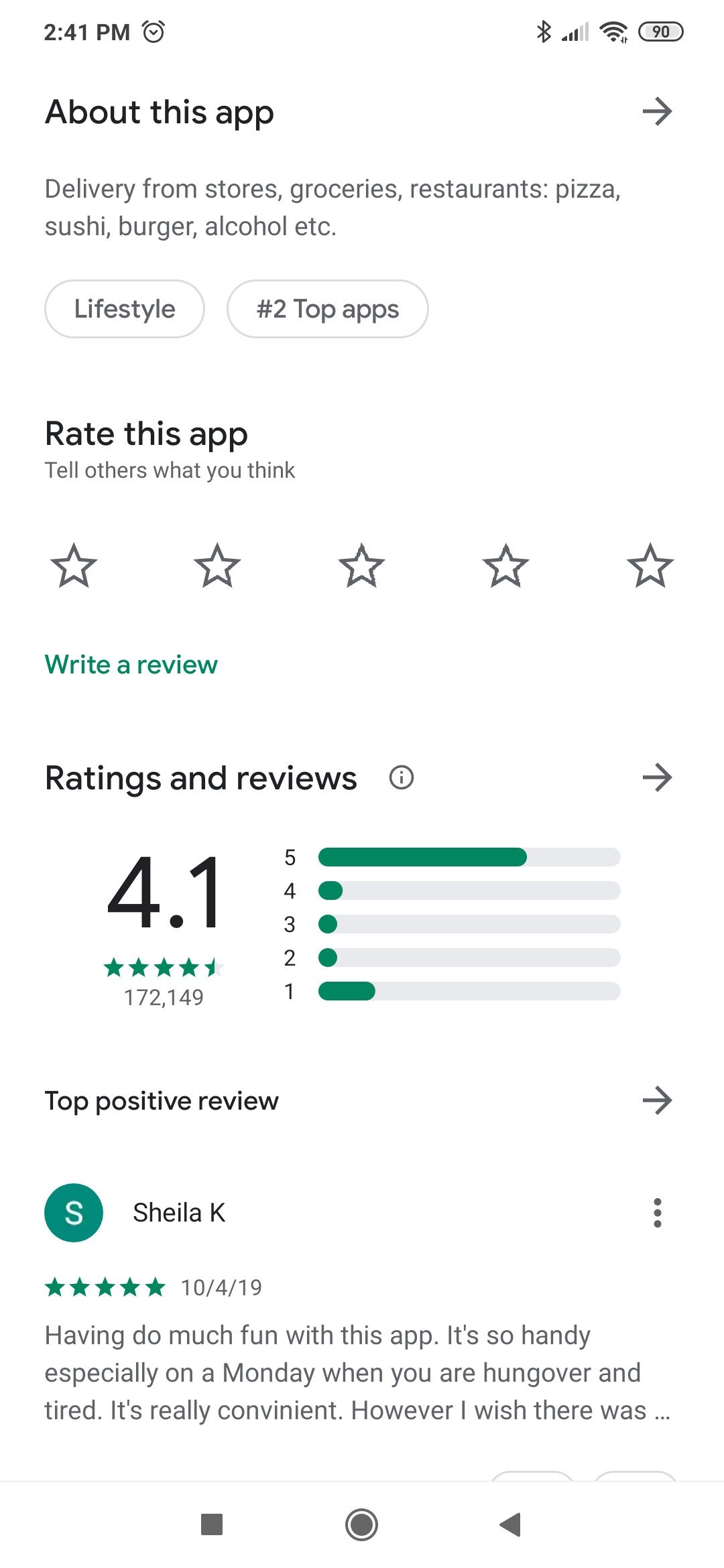This screenshot from a mobile phone displays various informational elements organized in a user-friendly interface. At the top left corner, the time and an alarm icon are visible, while on the right side, icons for Bluetooth, signal strength, Wi-Fi, and battery level are displayed. Below this, a heading reads "About this app" in black letters, followed by a description listing the app's services, including delivery from stores, groceries, restaurants, offering pizzas, sushi, burgers, alcohol, and more.

Further down, the interface shows categories under "Lifestyle" and the number two ranking among top apps. Users are prompted with the text "Rate this app, tell others what you think" above a line of horizontal stars for rating purposes. Additionally, there is a green hyperlinked text labeled "Write a review."

Underneath, a section titled "Ratings and Reviews" includes an arrow on the right side to access detailed reviews. The app has a rating of 4.1, displayed to the left of a bar graph that visually represents the distribution of ratings from one to five stars. Below this, there is a section for the "Top positive review," accompanied by an arrow pointing right. At the bottom of the screenshot, the review from the top positive reviewer along with their username can be seen.